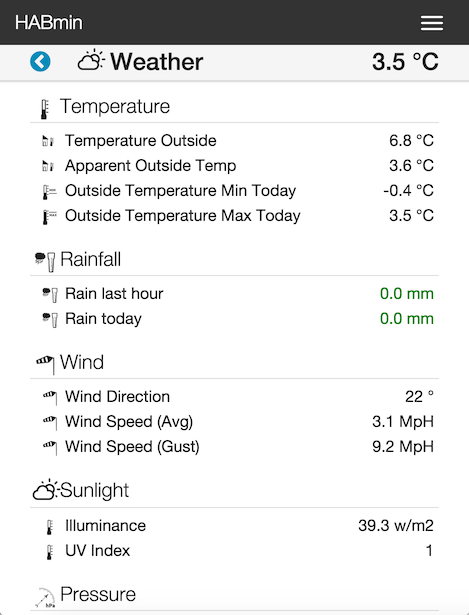The displayed webpage, accessible on both computers and mobile devices, is from "HAB Min." At the top, a black navigation bar contains the site name and a menu icon represented by three horizontal lines on the right side. Immediately below, a light gray strip runs across the screen, indicating weather information.

An icon showcasing a cloud and sun duo is prominently displayed. Adjacent to it, a blue circle with a leftward-pointing arrow features the temperature: 3.5 degrees Celsius. Below, the section elaborates with further details alongside a thermometer icon:

- **Current Temperature**: 6.8°C
- **Apparent Temperature**: 3.6°C
- **Minimum Outside Temperature Today**: -0.4°C
- **Maximum Outside Temperature Today**: 3.5°C

In terms of precipitation, the page states:

- **Rainfall in the Last Hour**: 0 mm
- **Rainfall Today**: 0 mm

Wind information is detailed as follows:

- **Wind Direction**: 22°
- **Average Wind Speed**: 3.1 mph
- **Wind Speed Gust**: 9.2 mph

Moving on to sunlight data, depicted with another sun and cloud icon, the webpage notes:

- **Illuminance**: 339.3 W/m²
- **UV Index**: 1

However, no information is given under the "Pressure" section.